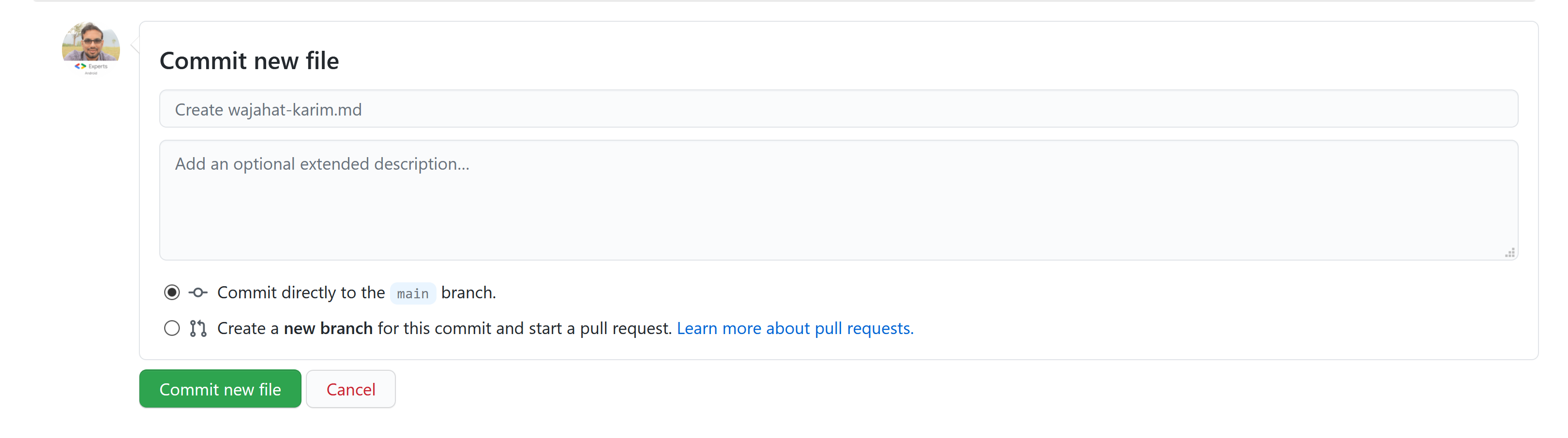This image provides a visual walkthrough of the process for creating a new file in a version control system. The central dialog box allows users to either commit directly to the existing branch or create a new branch for the commit and subsequently start a pull request. 

- On the left side of the image, a visual element features a Caucasian male, indicative of either a user icon or a guidance figure. 
- The dialog box prominently displays the option to "Commit new file" at the top. 
- Beneath this heading, there's a text input labeled "Create WAPT CARIM MD" and an additional field for an optional extended description.
- Users are given the choice to commit directly to the current branch or to create a new branch for their changes, supported by a separate link to "Learn more about pull requests" for further information.
- Crucial action buttons include "Commit new file" in a clickable green box, and a "Cancel" button in red letters within a white box, allowing users to back out if needed.

Overall, while the layout aims to guide users through these actions, it may appear confusing to those unfamiliar with the process, suggesting a need for clearer instructional support.